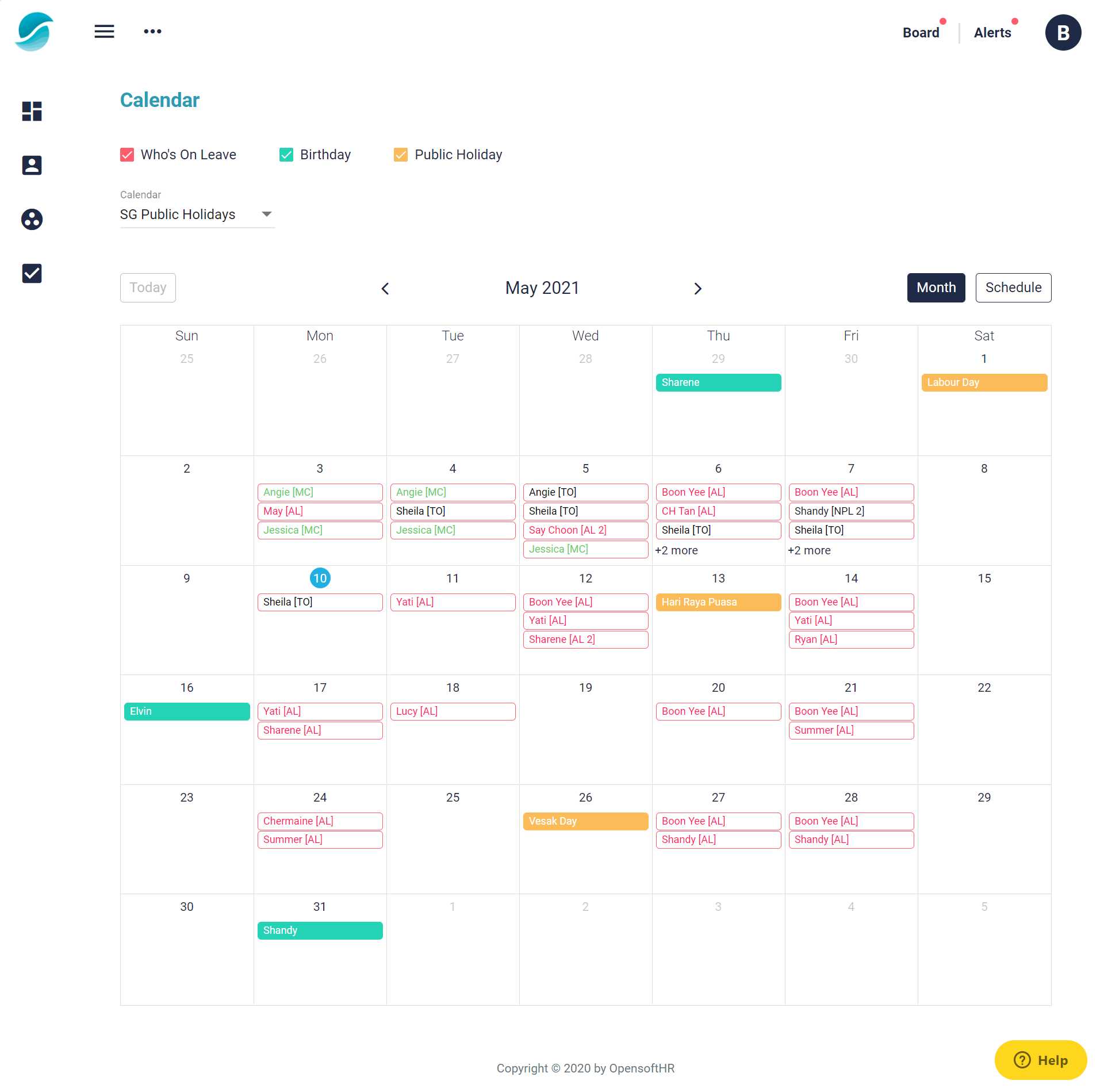This is a detailed screenshot of a calendar website, focused on the month of May 2021, displaying various events and holidays. The primary section features a traditional calendar layout, labeled "Calendar". According to the legend, red highlights indicate individuals on leave, green highlights signify birthdays, and yellow highlights denote public holidays. The calendar is currently set to display "SG Public Holidays." A dropdown menu is present for additional configuration options.

On the top right side of the interface, a black button is toggled to "Month," indicating the current view format, with an option to switch to a "Schedule" format. Specific names are highlighted in green to mark birthdays, including Shireen on Thursday, Elvin on the 16th, and Shandy on the 31st. Numerous entries in red presumably show individuals on leave, while yellow cells mark significant public holidays such as Labor Day on May 1st, Hari Raya Puasa on May 13th, and Vesak Day on May 26th. Additionally, there is a yellow help button located in the bottom right corner of the screen for user assistance.